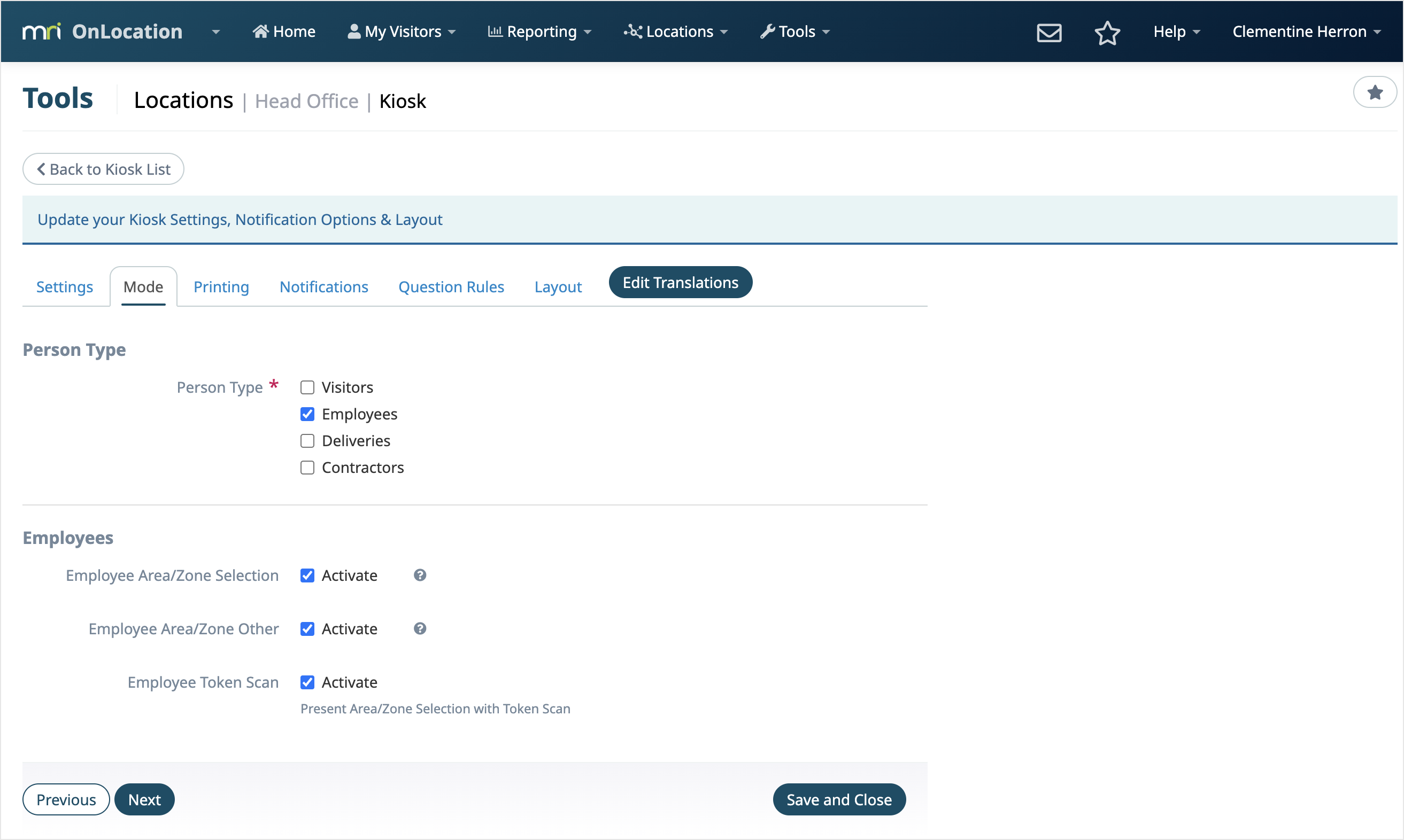The webpage presents a well-organized interface for MRI's "On Location" application, characterized by clarity and essential functionalities. At the top, a white-green-white logo spells out "MRI," adjacent to the title "On Location." 

The navigation bar categorizes content into sections such as Home, My Visitors, Reporting, Location, and Tools. On the top-right corner, you find icons for Mail, Favorites, Help, and a user name: Clementine Heron.

Within the Tools section, there is a hierarchical structure featuring Locations, with subsections like Head Office and Kiosk. A conspicuous button labeled "Back to Kiosk List" facilitates navigation. Below is an area titled "Update your Kiosk Settings," offering various options like Notification Options and Layouts.

Users can configure an extensive range of settings, including Settings, Mode, Printing, Notifications, Question Rules, Layouts, and Edit Translations. The "Person Type" field is marked with an asterisk and features checkboxes for Visitors, Employees, Deliveries, and Contractors, with only the Employees checkbox selected.

The Employees section encompasses subsections such as Employee Area/Zone Selection, Employee Area Zone/Other, and Employee Token Scan, all of which are activated. At the bottom, action buttons include a white "Previous" button, a darker gray "Next" button, and a gray "Save and Close" button.